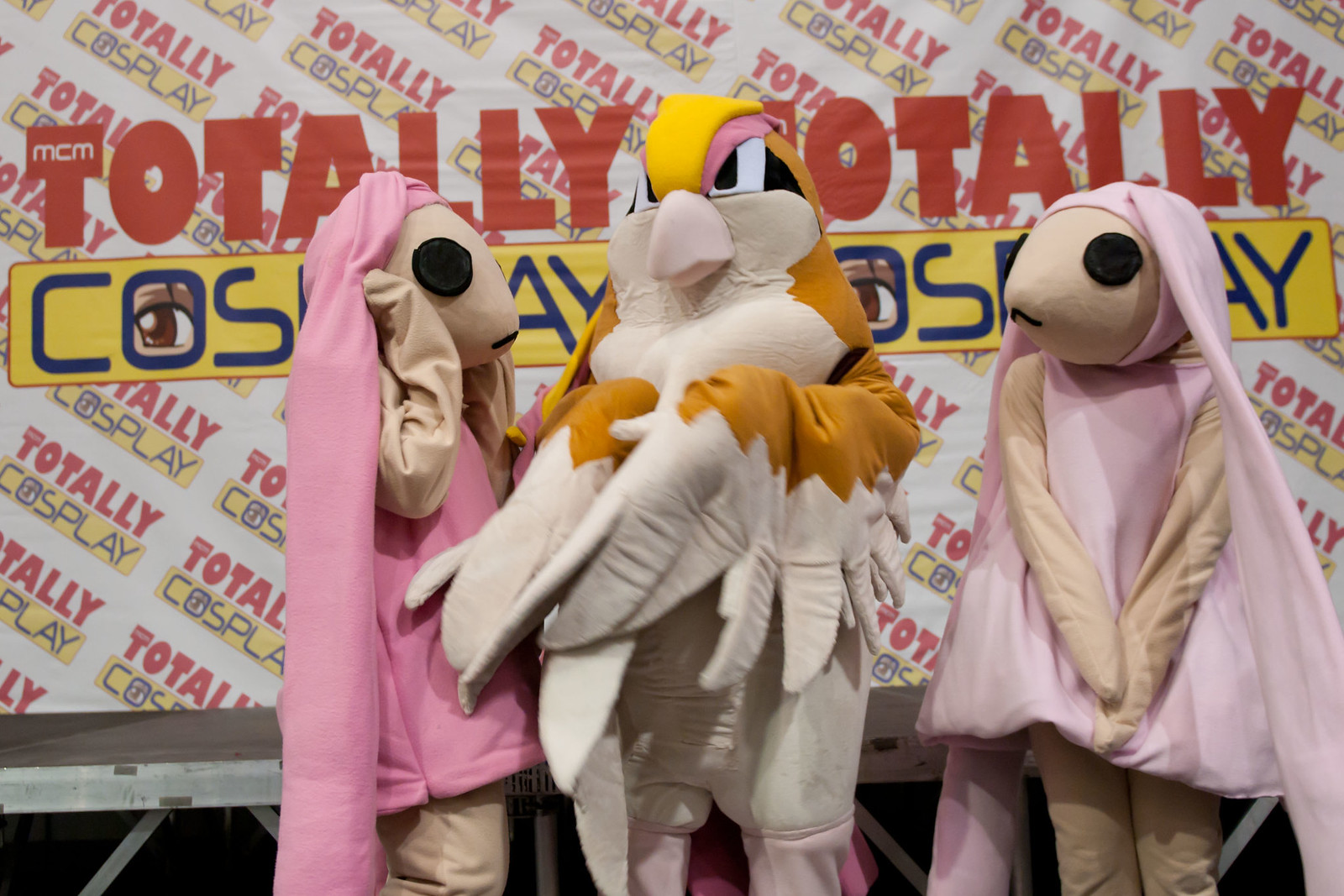Three individuals are standing at a cosplay convention, posing in elaborate animal costumes against a backdrop with the banner "Totally Cosplay MCM." The central figure is dressed as a bird, featuring a large costume with a cream-colored base, light brown accents, and striking yellow feathers. The bird costume has a distinct gray or cream-colored beak, expressive black-and-white eyes, some pink highlights, and an overall detailed design. On the right, a figure is dressed as a rabbit, characterized by long floppy ears, black eyes, a simple black mouth, and a bright pink dress. The setting appears to be indoors, possibly on a stage or at a red carpet event, with vivid colors including white, red, yellow, blue, pink, black, and brown that add vibrancy to the scene.